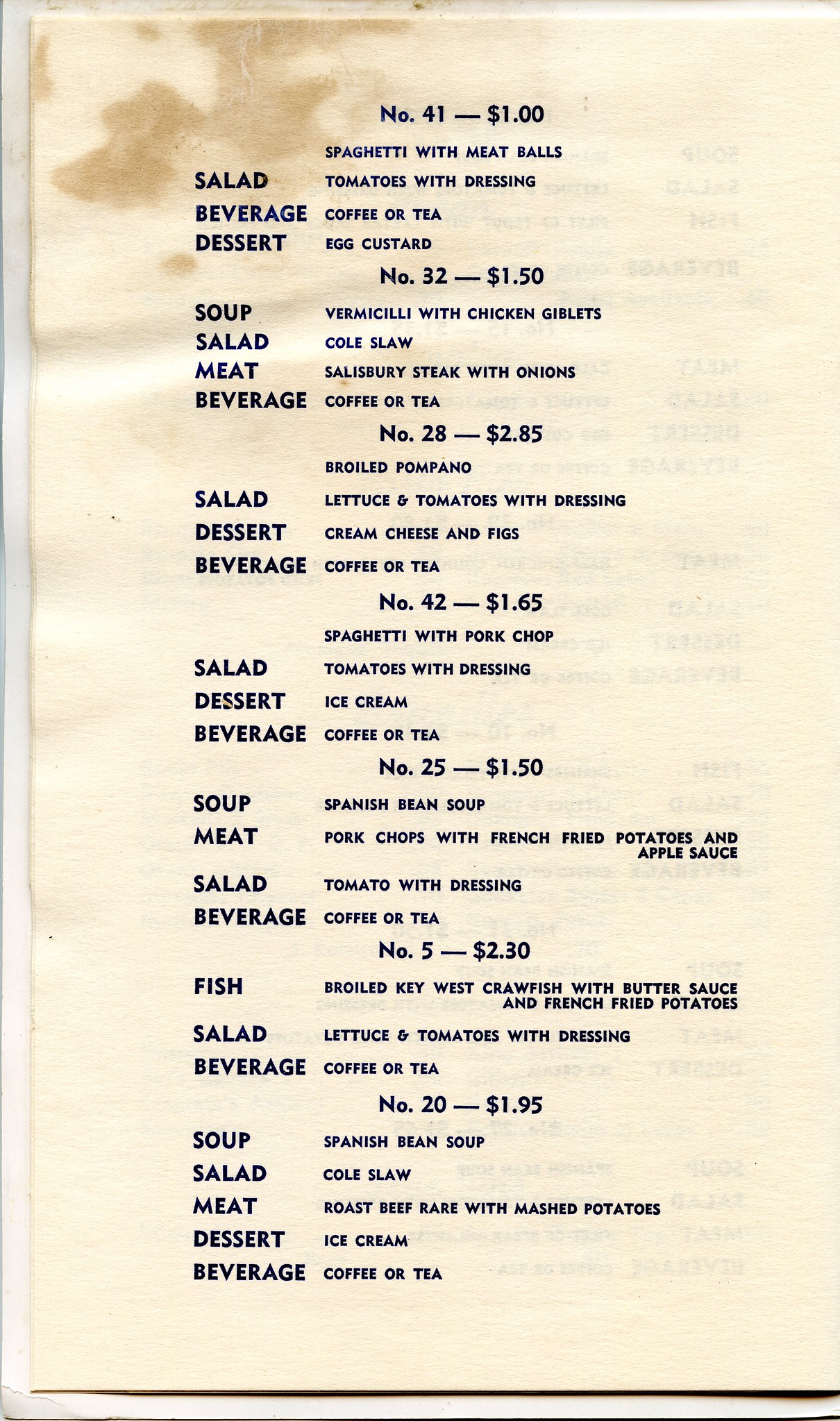This image depicts a vintage menu page, heavily yellowed with age, suggesting it dates back to the 1970s or 1980s, if not earlier. The page has suffered water damage, evident from its curling left-hand side and a noticeable stain at the top corner that may be from water or coffee. The page lists several meal options, each accompanied by surprisingly low prices reflective of the era. The offerings are as follows:

- **Menu Item No. 41**: $1.00 – *Spaghetti with meatballs, salad (tomatoes with dressing), beverage (coffee or tea), dessert (egg custard).*
- **Menu Item No. 32**: $1.50 – *Soup (vermicelli with chicken giblets), salad (coleslaw), Salisbury steak with onions, beverage (coffee or tea).*
- **Menu Item No. 28**: $2.85 – *Broiled pompano, salad (lettuce and tomatoes with dressing), dessert (cream cheese and figs), beverage (coffee or tea).*
- **Menu Item No. 42**: $1.65 – *Spaghetti with pork chop, salad (tomatoes with dressing), dessert (ice cream), beverage (coffee or tea).*
- **Menu Item No. 25**: $1.50 – *Soup (Spanish bean soup), pork chops with French fried potatoes and applesauce, salad (tomato with dressing), beverage (coffee or tea).*
- **Menu Item No. 5**: $2.30 – *Broiled Key West crawfish with butter sauce and French fried potatoes, salad (lettuce and tomatoes with dressing), beverage (coffee or tea).*
- **Menu Item No. 20**: $1.95 – *Soup (Spanish bean soup), salad (coleslaw), roast beef (rare) with mashed potatoes, dessert (ice cream), beverage (coffee or tea).*

The menu displays a variety of choices, although not in any particular order. The thinness of the paper allows a glimpse of additional menu items printed on the reverse side.